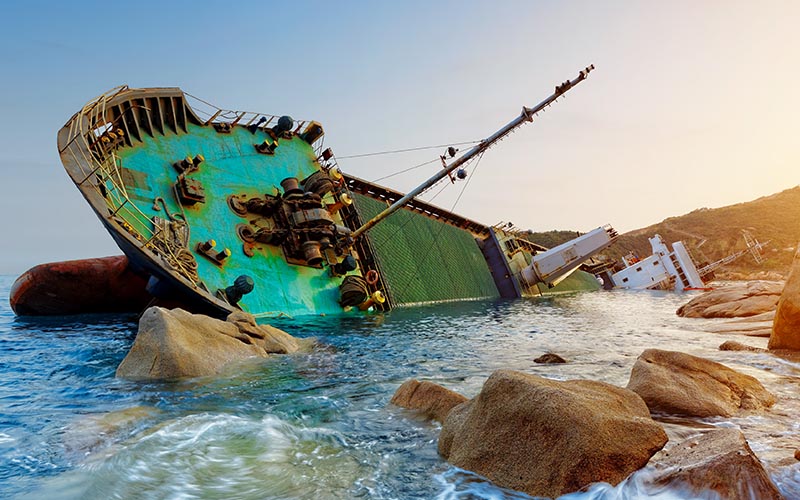The image depicts a large ship in a precarious position, seemingly leaning on its side near a rocky coastline under a sunlit sky that suggests it's either sunset or sunrise, with a slight haze on one side of the horizon. The ship, which is devoid of any visible human presence, appears to be in distress, leaning at an angle with its bridge and portions clearly visible. It looks dangerously close to submerging, half-submerged already, and the deck of the first floor is covered in rust and green oxidation, indicative of prolonged exposure to the elements. The ship’s angle reveals its two diagonal flagpoles prominently. The setting is tranquil yet starkly juxtaposed with the ship's chaotic state, accentuated by the sunlight casting a warm glow over the scene. In the distant horizon to the right, land is visible, emphasizing the nearness to the coastline. The overall impression suggests a possible shipwreck or an art installation meant to evoke such a scene.